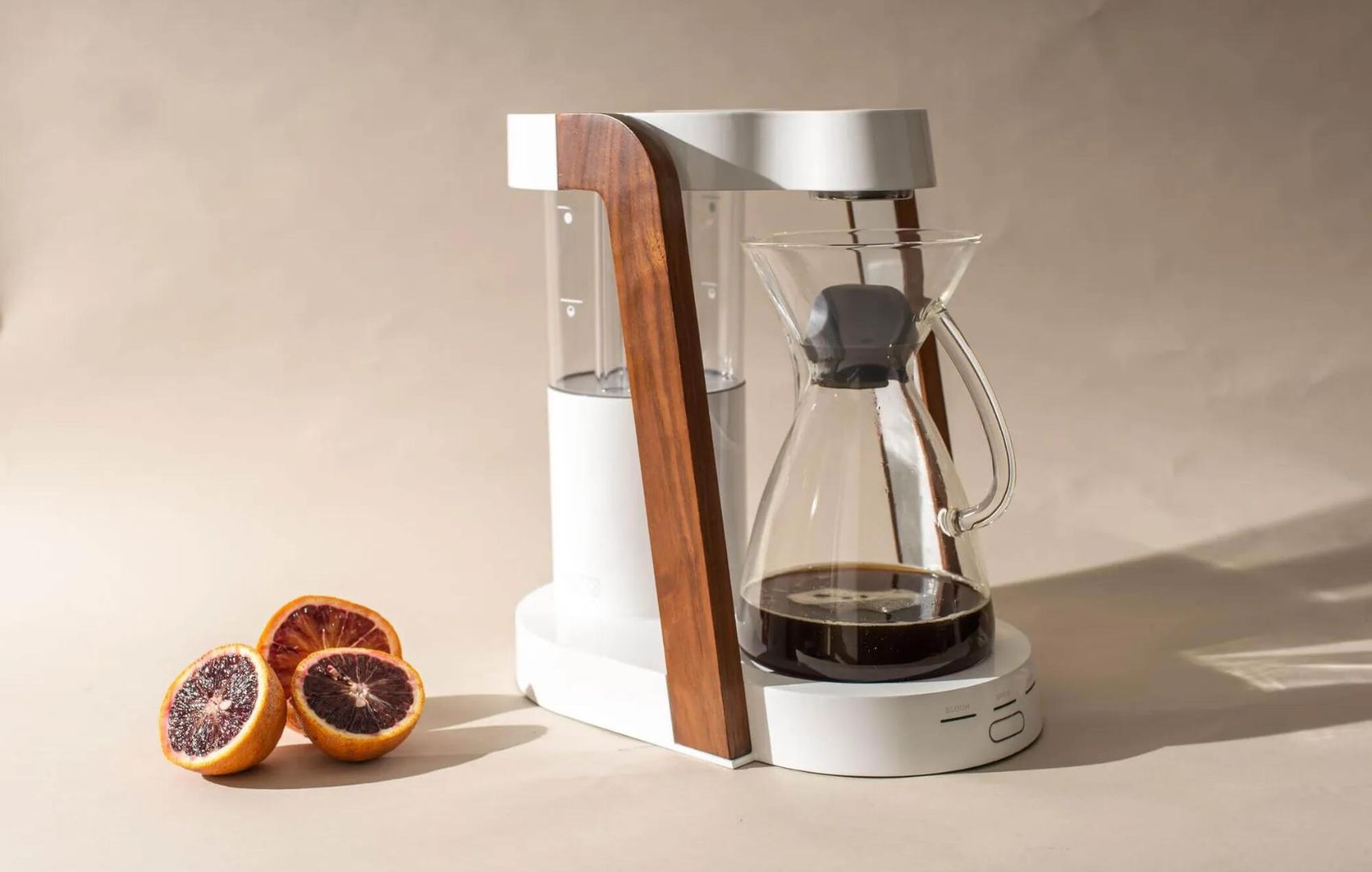The image features a sleek, Nordic-style coffee machine set against a light, beige-tan background. The coffee machine has a white base with elegant wooden trims along the sides and a white top. It includes an hourglass-shaped glass pitcher with a curved handle, partially filled with freshly brewed coffee. On the left side of the image, there are three halves of a blood orange, showcasing a striking dark red center encircled by a white ring, and orange peel. The setup appears to be part of a professional product photo shoot, highlighted by the soft shadows cast by both the coffee machine and the fruit.